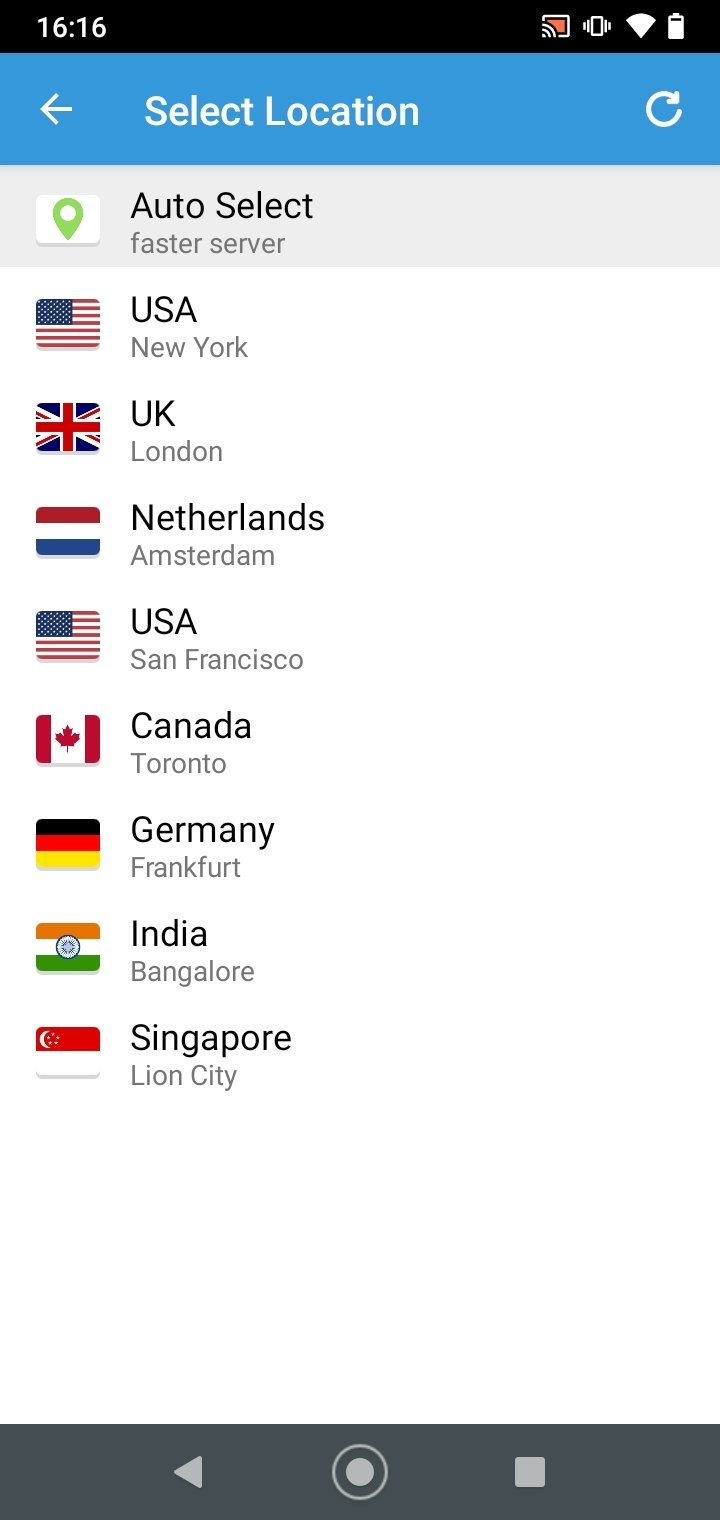This image is a detailed screenshot of a cellular phone screen taken at 4:16 PM. The phone is connected to Wi-Fi, set to vibrate mode, and the battery is almost fully charged, as indicated by the icons in the upper right corner. The user is casting their screen onto a television. 

At the top of the screen, under a light blue bar, are UI elements including a back arrow pointing left, the text "Select Location," and a refresh icon on the far right. Below this bar, in black text, it says "Auto Select Faster Server," accompanied by a green location icon.

The screen lists multiple server locations with their respective flags and names:
- USA, New York
- UK, London
- Netherlands, Amsterdam
- USA, San Francisco
- Canada, Toronto
- Germany, Frankfurt
- India, Bangalore
- Singapore, Lion City

At the very bottom, there is a gray navigation bar featuring a back arrow, a home button circle, and a square icon for toggling between apps on the right side.